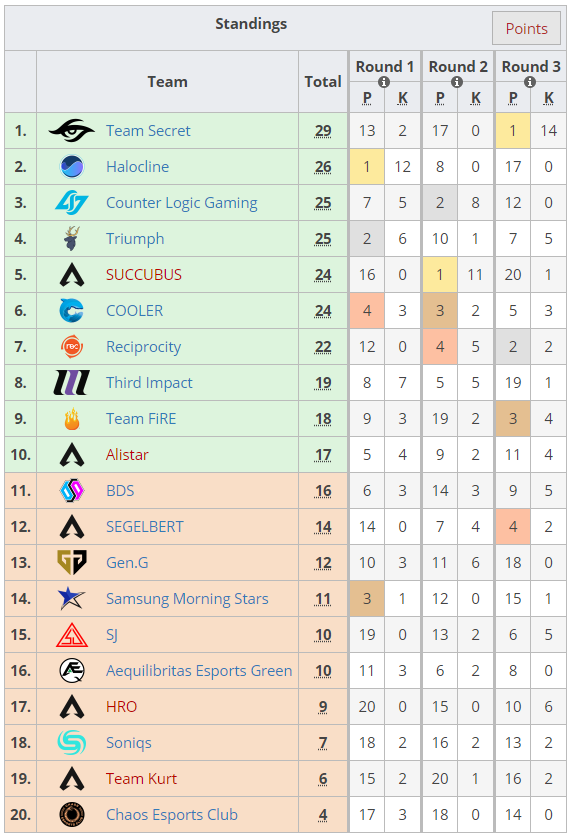The image showcases a detailed standings chart for a tournament, with various columns providing specific statistics. At the top, the chart is labeled "Standings". The chart is divided into sections with columns titled "Points" on the right, "Teams" next to it, followed by columns for "Total", and rounds "1 PK", "2 PK", and "3 PK".

The rankings are displayed vertically from numbers 1 to 20. Each team is listed with its logo on the left side of their name.

1. **Team Secret** is ranked number one with a total of 29 points. Round 1 has 13 points (13p) and 2 kills (2k), Round 2 has 17 points (17p) and 0 kills (0k), and Round 3 has 1 point (1p) and 14 kills (14k).
2. **Halo Klein** stands in second place with a total of 26 points. Round 1 has 1 point (1p) and 12 kills (12k), Round 2 has 8 points (8p) and 0 kills (0k), and Round 3 has 17 points (17p) and 0 kills (0k).
3. **Counter Logic Gaming** is in third place with a total of 25 points. Round 1 has 7 points (7p) and 5 kills (5k), and Round 2 has 8 points (8p) and 0 kills (0k).

Overall, the table provides a clear overview of the performance of the top teams across different rounds, emphasizing their point totals and kill counts per round.